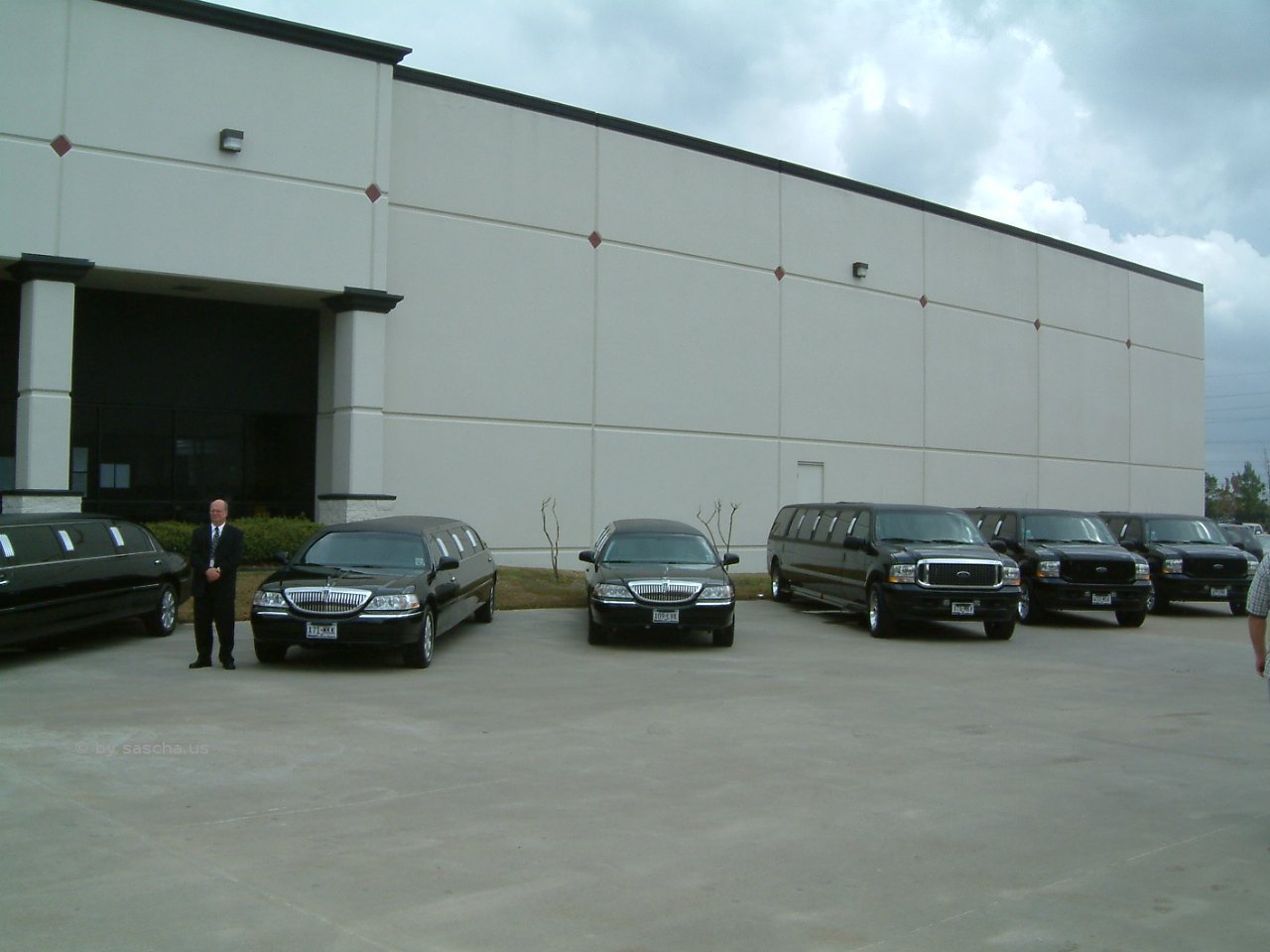The photograph captures a fleet of extended black limousines, including Lincoln and Ford models, lined up in front of a modern, one-story industrial-style white building with a light gray exterior. The building features several square grid lines and light landscaping, including a hedge near a prominent arch entrance. The scene is set against a sky with puffy storm clouds gathering in the top right corner. On the foreground pavement, a well-dressed gentleman in a black suit, dark tie, and white shirt stands with his hands folded in front of one of the limousines, adding a touch of formality to the setting. The overall impression suggests a limousine dealership or rental service. An isolated left arm of a passerby can be seen towards the left-center of the image.